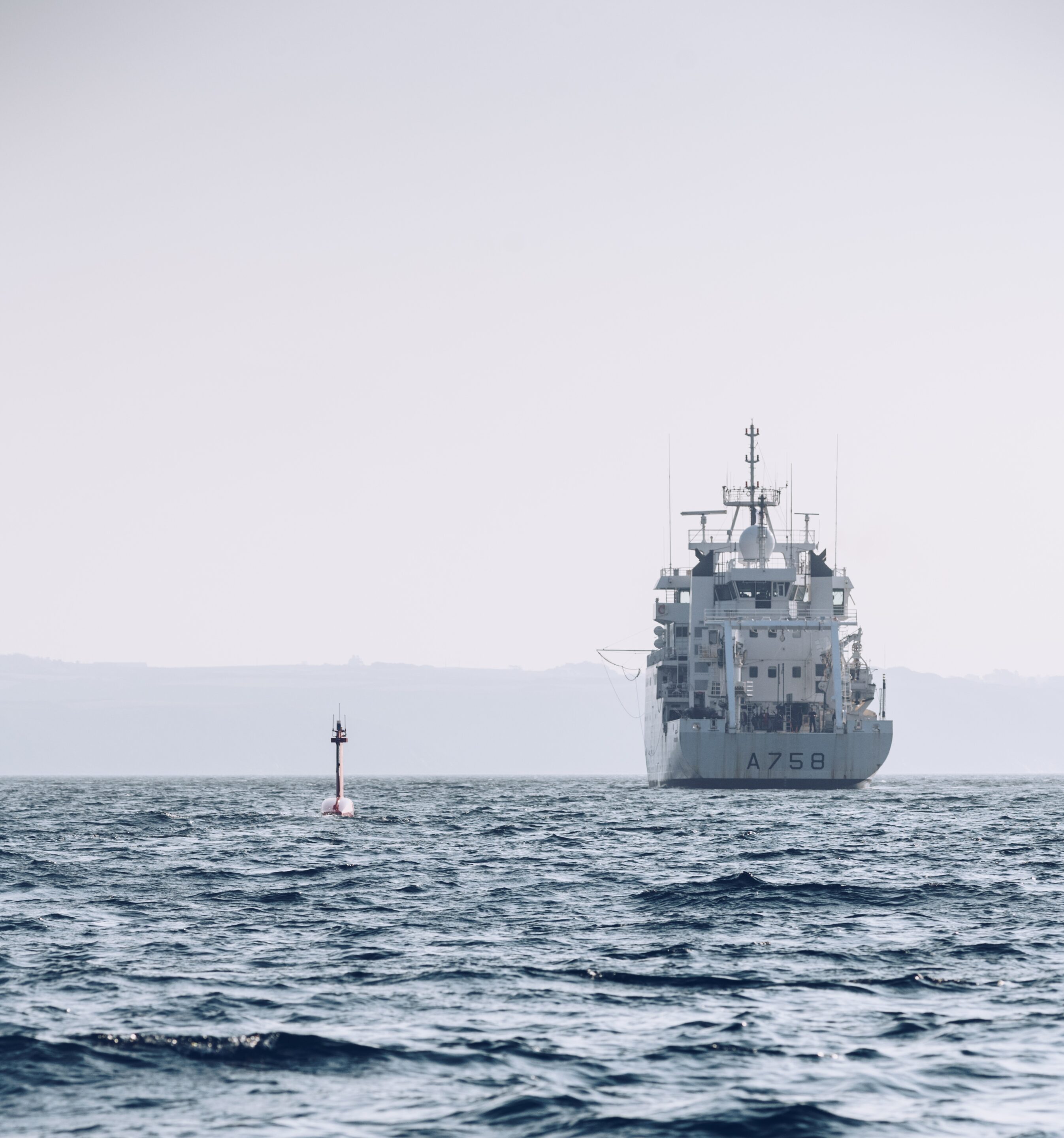The image depicts a large, multi-level battleship navigating through calm, dark blue waters, though the overall tone appears gray and hazy due to fog. The ship, labeled with the designation A758, features several satellites and antennae, a large round structure on top, and an area where people are likely conducting operations. To the left of the ship, a white buoy with some orange paint is visible. In the distant background, a series of interconnected, hazy mountains stretch along the horizon, hinting at a foggy, indistinct sky. The ship seems equipped with small emergency boats hanging off its right side and appears to be heading towards the observer.